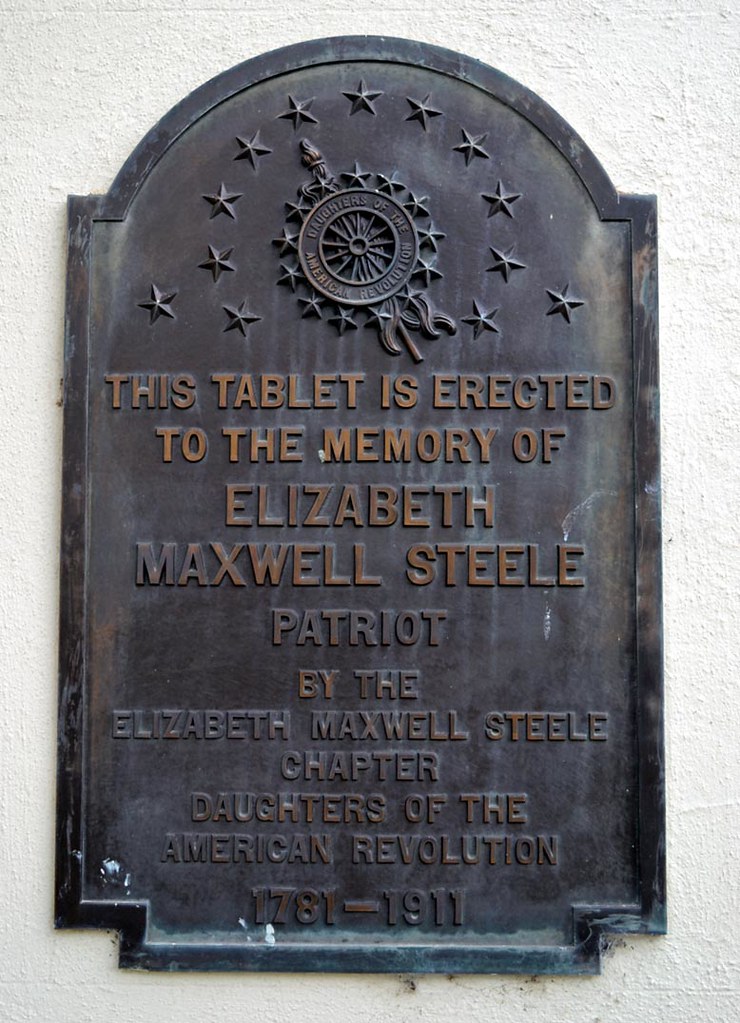This image depicts a rectangular metal plaque, likely made from iron or copper, affixed to a wall or potentially part of a statue. The plaque has a rounded top and features raised, embossed lettering. At the very top, there are thirteen stars arranged in a circular pattern. Within this circle, there is an insignia, although it appears somewhat worn and difficult to read due to patina covering much of the plaque's surface.

The main text of the plaque reads: "This tablet is erected to the memory of Elizabeth Maxwell Steele, patriot, by the Elizabeth Maxwell Steele chapter, Daughters of the American Revolution." Below this dedication, the dates "1781 to 1911" are inscribed. Despite the patina obscuring part of the plaque, the inscription remains legible.